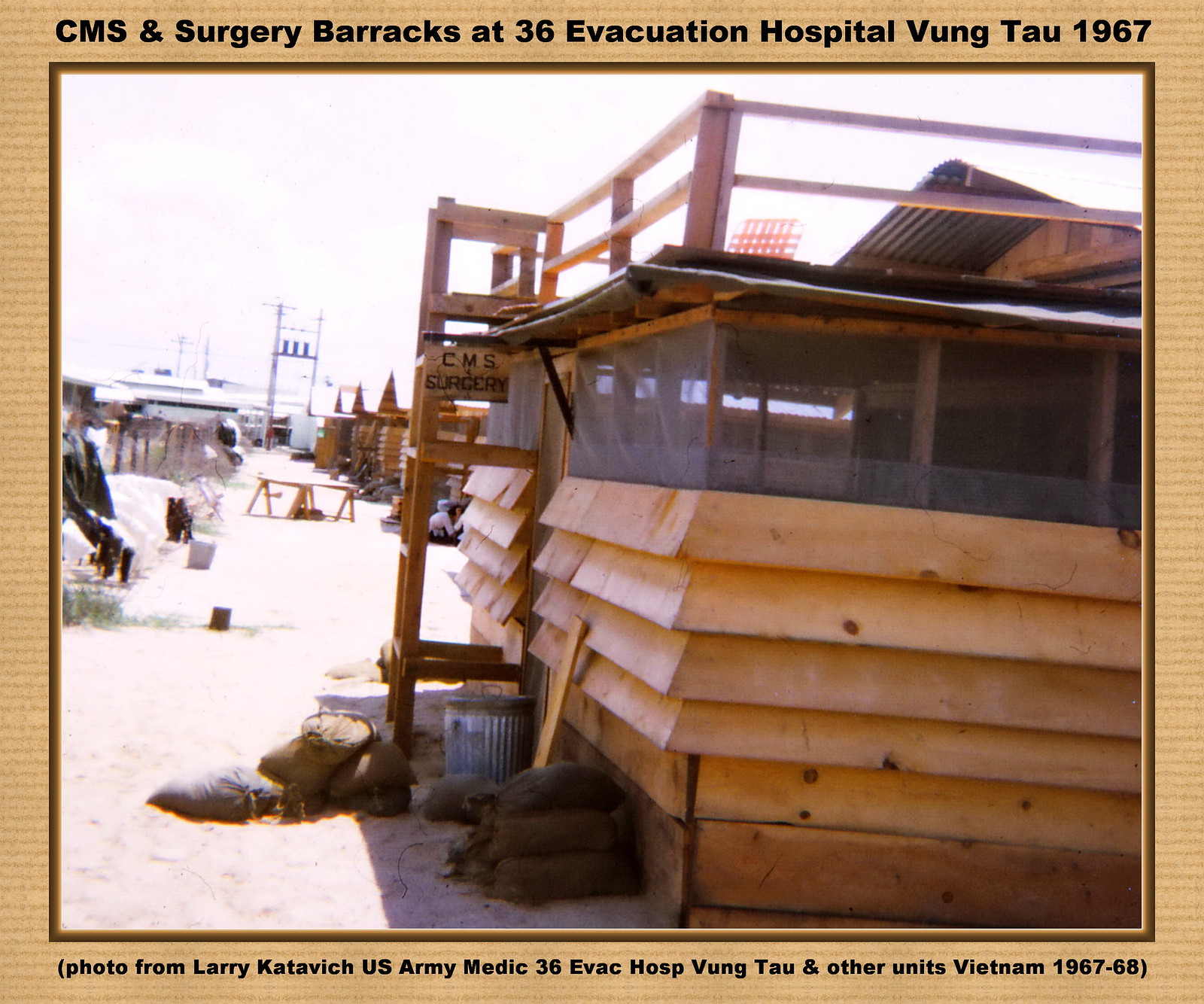This vintage color photograph from 1967, labeled at the top "CMS and Surgery Barracks, 36 Evacuation Hospital, Vung Tau, 1967," showcases a simple one-story wooden building with mesh-net windows and a corrugated roof. A ladder on the side allows access to the roof, and sandbags flank the left of the structure. The photograph's border mimics light brown wood with a textured finish, and additional text at the bottom reads "Photo from Larry Katovich, U.S. Army Medic, 36 Evac Hospital, Vung Tau, and other units, Vietnam, 1967-1968." The building, along with other similar shacks, is built on a sandy stretch under a bright white sky, indicative of the harsh, bright sunlight. Power lines are visible, emphasizing the wartime setting. The image highlights not only the physical environment but also the everyday aspects of life at an evacuation hospital during the Vietnam War.